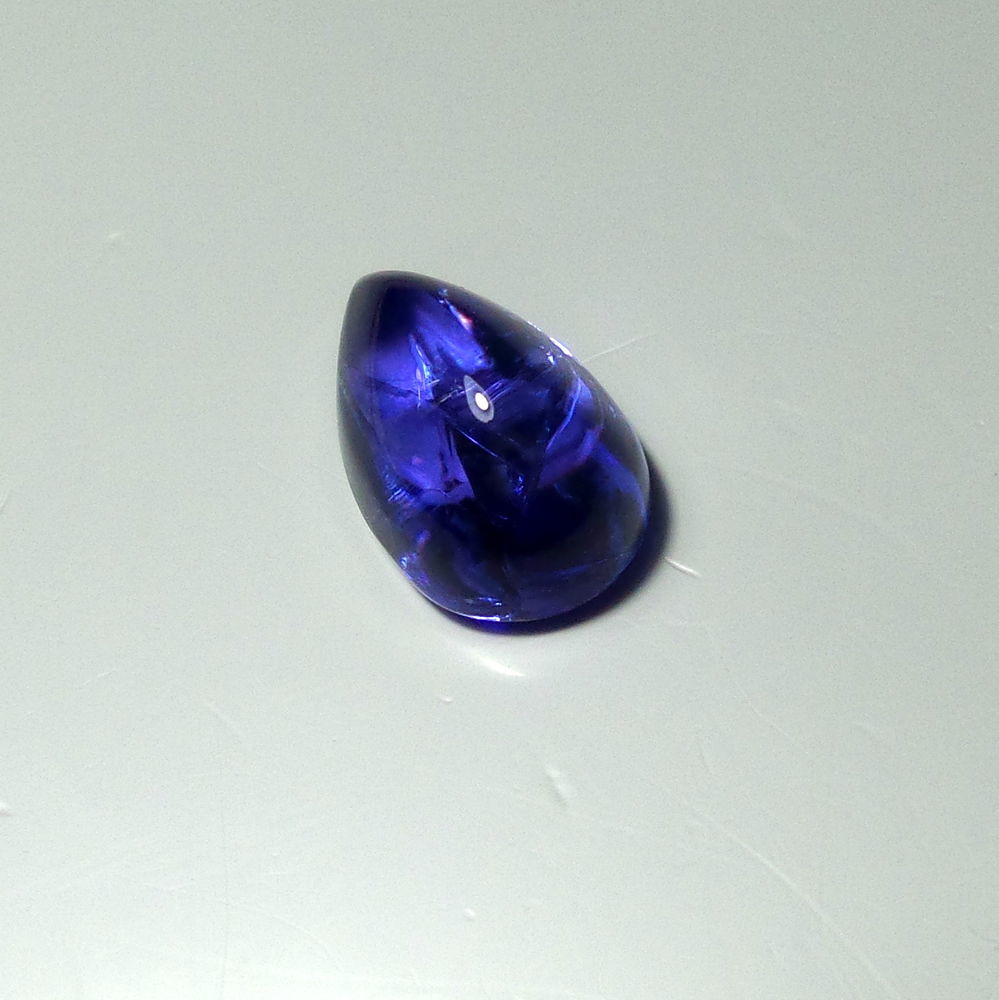The photograph features a highly polished, teardrop-shaped stone that is mostly deep blue with shades of black. The stone is positioned on a white, flat surface that appears somewhat soft, exhibiting numerous scratches and indents. The pointed end of the stone is directed towards the top left corner of the image, while the rounded bottom faces the bottom right. Notably, the stone’s reflective surface captures detailed reflections of its surroundings, including the person holding a phone to take the photograph and a light bulb overhead. Beneath the stone, a subtle shadow accents the lower right side, further highlighting its three-dimensional form against the potentially poster board-like background.